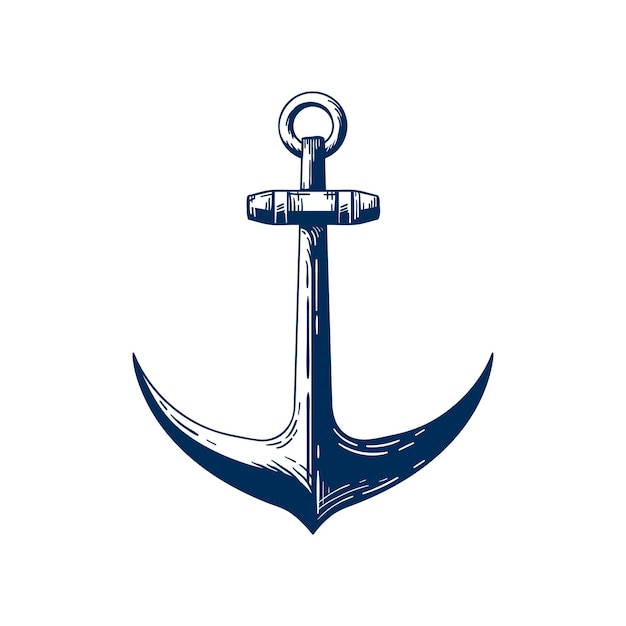This detailed illustration depicts an anchor rendered in dark blue and white shades, standing upright against a plain white background. The left side of the anchor is predominantly white, while the right side features a darker blue color, with additional shading at the bottom to enhance the sense of depth. At the top of the anchor, there's a large ring designed for threading a rope through. Just below this ring, a horizontal bar, pointed at both ends, extends across the anchor and exhibits signs of wear and tear, featuring subtle details of scratches and crosshatching. The anchor's base tapers to a point, completing its traditional shape. Overall, the drawing is more detailed than an average sketch, incorporating intricate lines to suggest light and dimension.